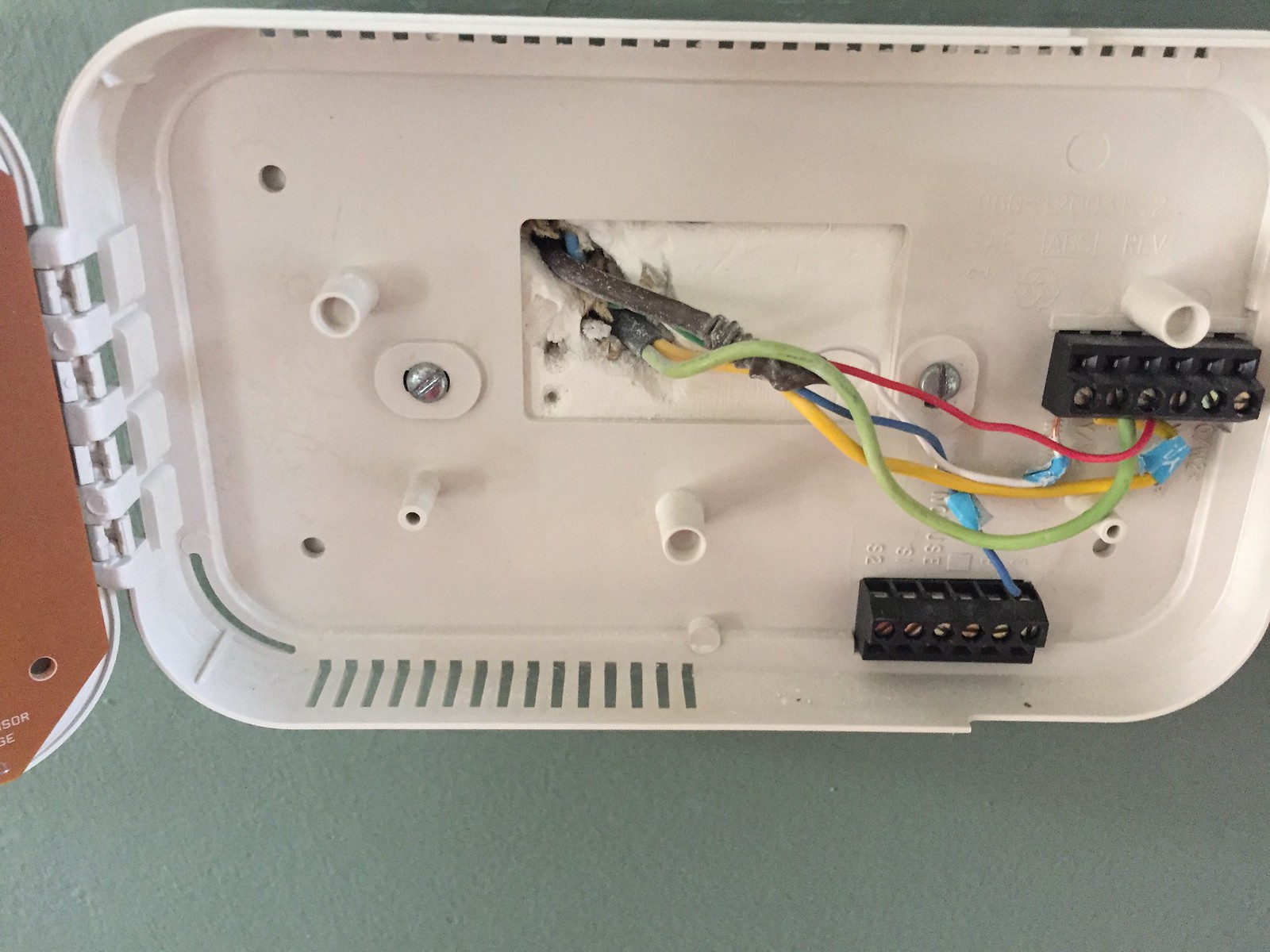Close-up image of an AC control panel or a similar device mounted either on a wall or ceiling, with an olive-gray background. The white compartment is open, with the door hinged on the left, revealing an intricate array of wires inside. Visible wires include green, blue, white, red, and yellow, originating from the back of the compartment and connecting to two black components within the device: one located to the right and the other at the bottom. The blue wire connects to the bottom black component, while the rest link to the right one. There are two screws securing the device to its mount, and a small vent is visible at the bottom left of the white compartment.